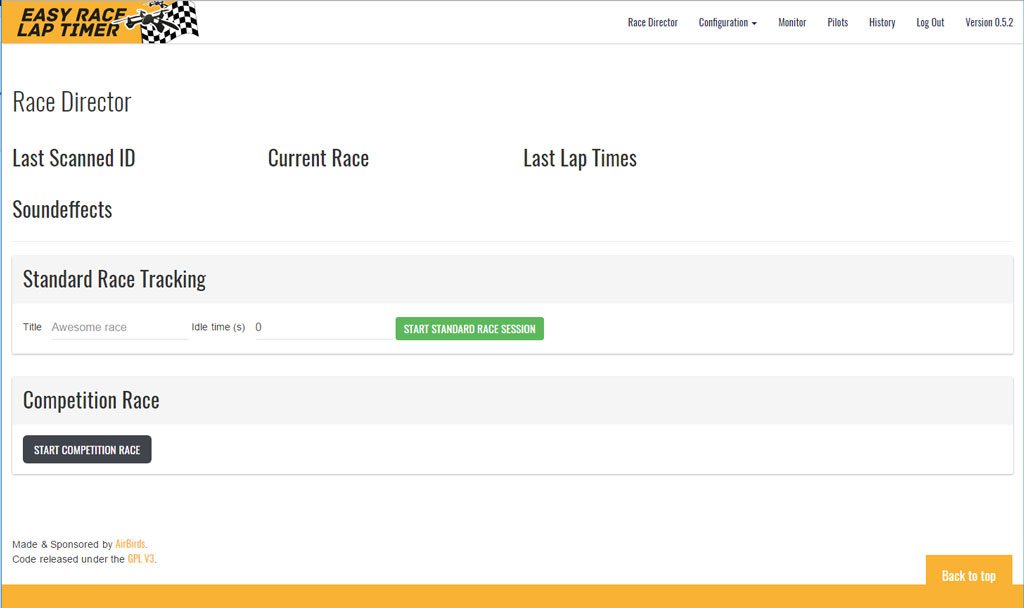**Screenshot of Easy Race Lap Timer Interface (Version 0.5.2)**

The image is a screenshot with a white background, showcasing the interface of the Easy Race Lap Timer. Prominently, at the top left corner, is a yellow rectangle with the text "Easy Race Lap Timer" in black. To the right of this label, there are options for "Race Director" and "Configuration."

The interface allows users to monitor various aspects such as the pilot's history and offers a logout option. The current version of the software is indicated as 0.5.2.

The "Race Director" section includes several functionalities:
- Last Scan ID
- Current Race
- Last Lap Times
- Sound Effects
- Standard Race Tracking Title 

Beneath these headings, there's a label for "Awesome Race" and a field titled "Idle Time (s)" which currently shows a value of 0. 

Highlighted in a green rectangle is the option to "Start Standard Race Session." Next to it, a black rectangle with white text provides the option to "Start Competition Race."

At the bottom left corner, the interface acknowledges its sponsors and creators with the text "Made and Sponsored by AvBets," where "AvBets" (spelled A-V-B-E-T-S) is in orange. Below this, it is mentioned that the code release is under the GPIV-3 license.

Lastly, at the bottom right corner, a yellow rectangle with white text offers a "Back to Top" option for easy navigation.